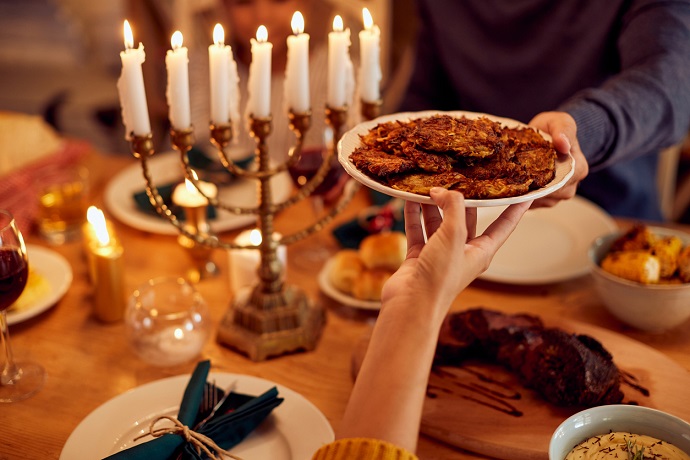The image features a formal dinner setting, likely a family gathering during the Jewish holiday of Hanukkah, as indicated by the prominent menorah at the center of the polished wooden table. The brass or gold menorah, adorned with seven lit white candles, stands as a focal point amidst an array of festive elements. A man, dressed in a black shirt, is seen passing a plate of food, possibly fried, to a woman who is partially visible, clad in a yellow or gold sweater. Beside the man, a blurred figure of a young girl in a white outfit suggests the presence of a child. The expansive table is teeming with dishes including meat, potatoes, corn on the cob, rolls, and possibly some soup. The place settings are meticulously arranged with plates accompanied by green and blue napkins, both neatly tied with twine. Additional candles and glasses of red wine add to the warm and inviting ambiance. The attention to detail extends to every element on the table, from the tied napkins to the embellishments on the potato dish, highlighting the care and celebration typical of a cherished holiday meal.